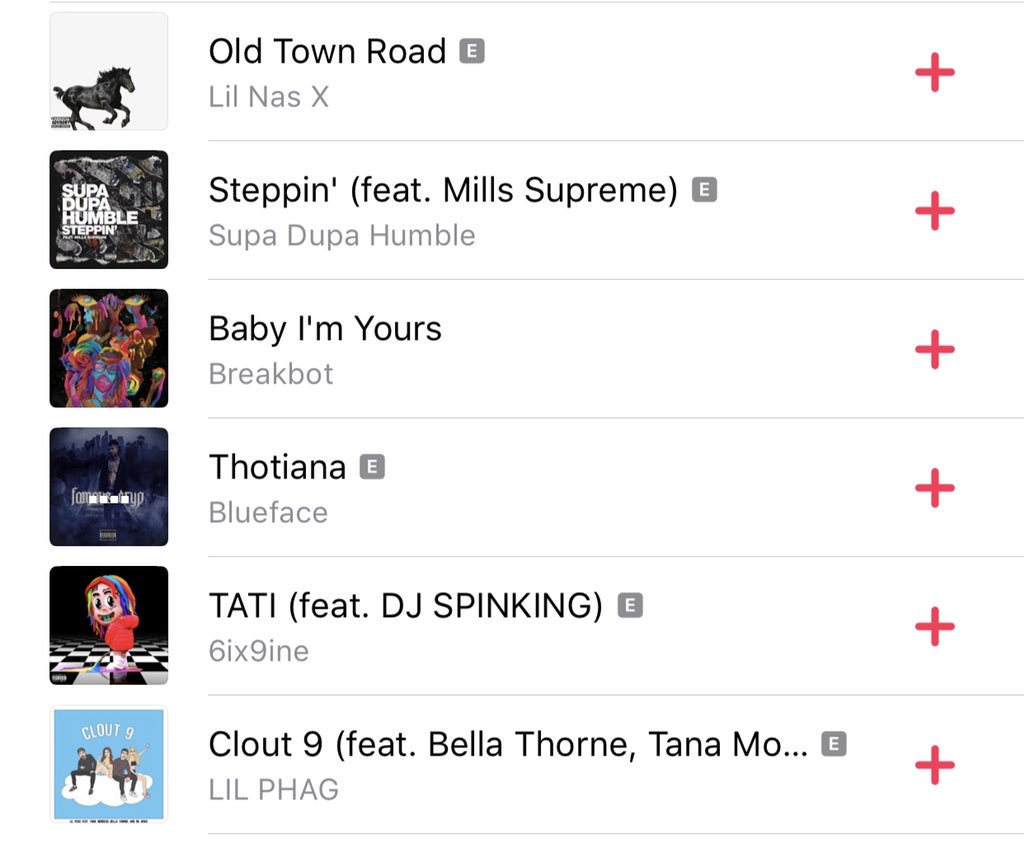This image showcases a selection of six different music tracks from various albums, likely displayed on a digital music platform where songs can be added to a playlist. Each track is accompanied by its respective album artwork, textual details, and a red plus sign indicating the option to add the song to a playlist. Thin gray lines separate each entry for clarity. Here's a detailed breakdown of the image content:

1. **Old Town Road by Lil Nas X:** The first entry features a galloping horse on a white background. This song title is labeled with an "E" for explicit content. Next to the title is the artist name "Lil Nas X" and a red plus sign for adding the track.

2. **Step In by Supa Dupa Humble featuring Mills Supreme:** The second album cover shows graphics related to "Supa Dupa Humble" and the song "Step In," which features Mills Supreme. This entry is marked explicit and also has a red plus sign.

3. **Baby I'm Yours by Breakbot:** The third album has a very colorful cover with shades of pink, blue, purple, and green. The title "Baby I'm Yours" and artist "Breakbot" are displayed, along with the red plus sign.

4. **Thotiana by Blueface:** The fourth album shows a dark blue and black image of a face partly obscured by clouds. The song "Thotiana" by Blueface is labeled explicit and includes the red plus sign.

5. **Tati by 6ix9ine featuring DJ Spinking:** The fifth entry has details about the song "Tati" by 6ix9ine, featuring DJ Spinking. It is also marked as explicit, with a red plus sign.

6. **Clout 9 featuring Bella Thorne and Tana Emo by Lil Phag:** The final entry pertains to "Clout 9" by Lil Phag, featuring Bella Thorne and Tana Emo. This song is explicit as well, and a red plus sign is present to add the track.

Overall, the image presents a diverse collection of explicit-content songs from various artists and albums, with vibrant and distinctive album artwork for each.